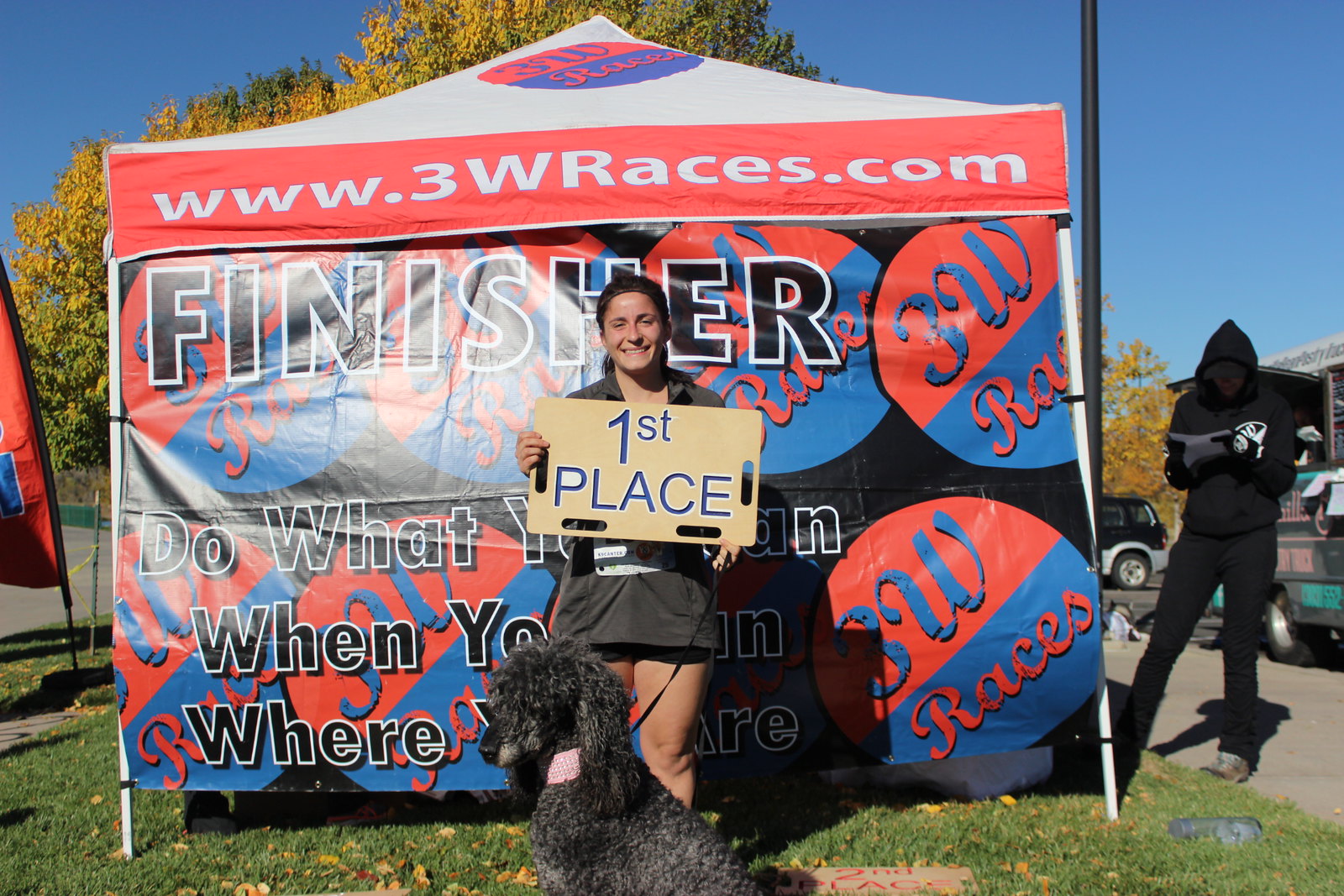In the image, a smiling woman with dark hair is proudly holding a tan-colored rectangular board marked with the words "FIRST PLACE" in bold blue letters. Dressed in a gray shirt and black shorts, she stands on a grassy area while holding the leash of a black poodle sitting obediently in front of her. Behind her, a large, partially visible colorful tent features a white top with a red vertical line displaying www.3wraces.com in white letters. The tent also has the word "FINISHER" in black letters outlined in white against half-red, half-blue circle designs. The background reveals a clear blue sky with some visible trees, vehicles, and a person dressed in all black, wearing a hoodie, and seemingly engrossed in a magazine.